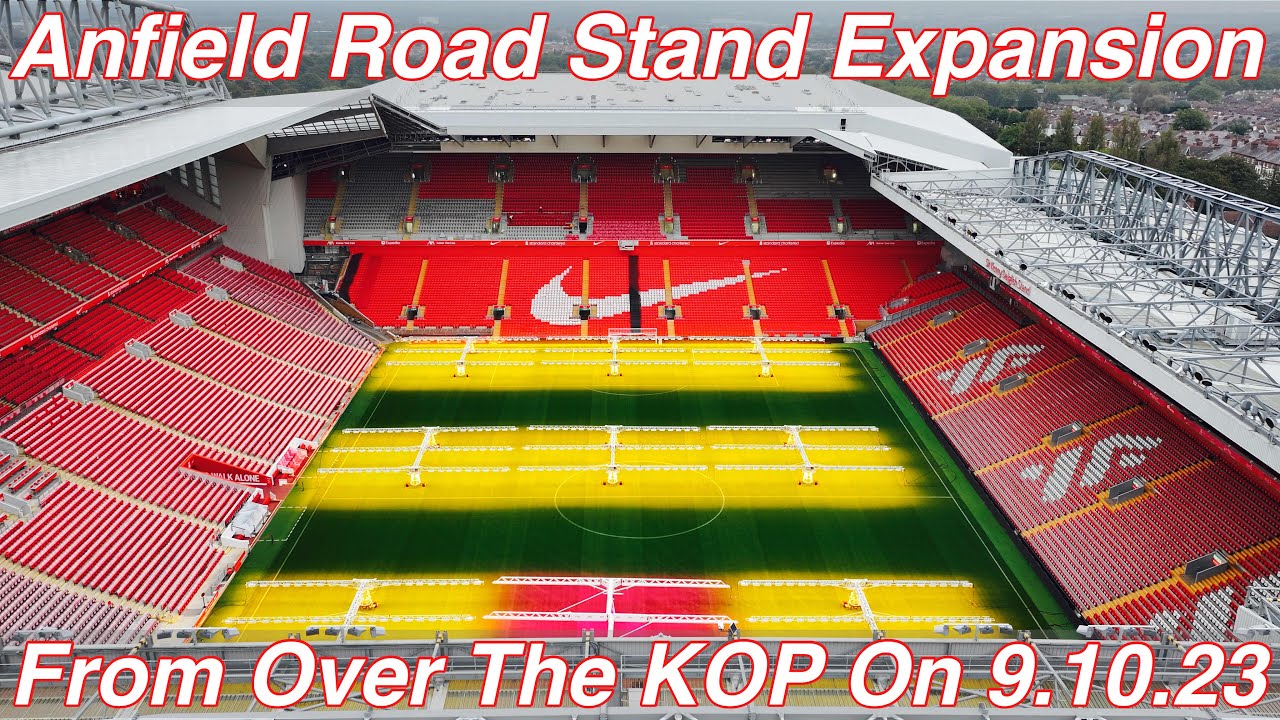The photograph captures a bird's-eye view of a large, empty soccer stadium, prominently featuring the text "Anfield Road Stand Expansion" at the top and "From over the KOP on 9-10-23" at the bottom. The picture is framed from an elevated angle above the KOP end, looking down towards the expansive field. The seats are predominantly red, with certain sections displaying a white Nike swoosh logo and some featuring orange stripes. The far end of the stadium, designated for the Anfield Road Stand, is partway through an expansion as indicated by the scaffolding and construction visible on the silver-colored roofs. The open roof design allows a partial view of a cloudy skyline, with hints of trees, buildings, and a white bridge toward the background. The field itself is striped with alternating thick yellow and green sections, and features various white markings and bracing. In summary, the photograph not only highlights the scale and current state of the stadium but also outlines the planned significant seating expansion with detailed annotations.